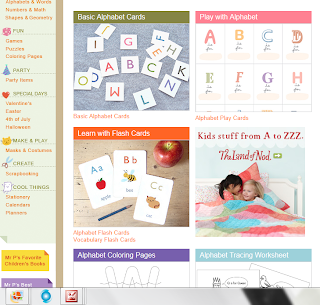This image appears to be a screenshot of a children’s educational website. On the left side of the webpage, there is a vertical menu bar, but the text within the menus is too small to be legible. To the right of this menu bar, the main content area is divided into four prominent tiles. 

- The first tile is titled "Basic Alphabet Cards" and features a picture of several colorful alphabet cards.
  
- The second tile is labeled "Play with Alphabet," accompanied by an image depicting alphabet cards as well.

- The third tile, "Learn with Flashcards," shows various educational flashcards beneath its title, indicating a focus on learning through visual aids.

- The fourth tile, "Kids Stuff from A to ZZZ," seems to suggest a collection of resources or activities, possibly including bedtime stories, as inferred from the playful 'ZZZ' in the title, symbolizing sleep.

Each tile appears to be a clickable link, guiding users to specific educational content geared towards young children’s learning and play.